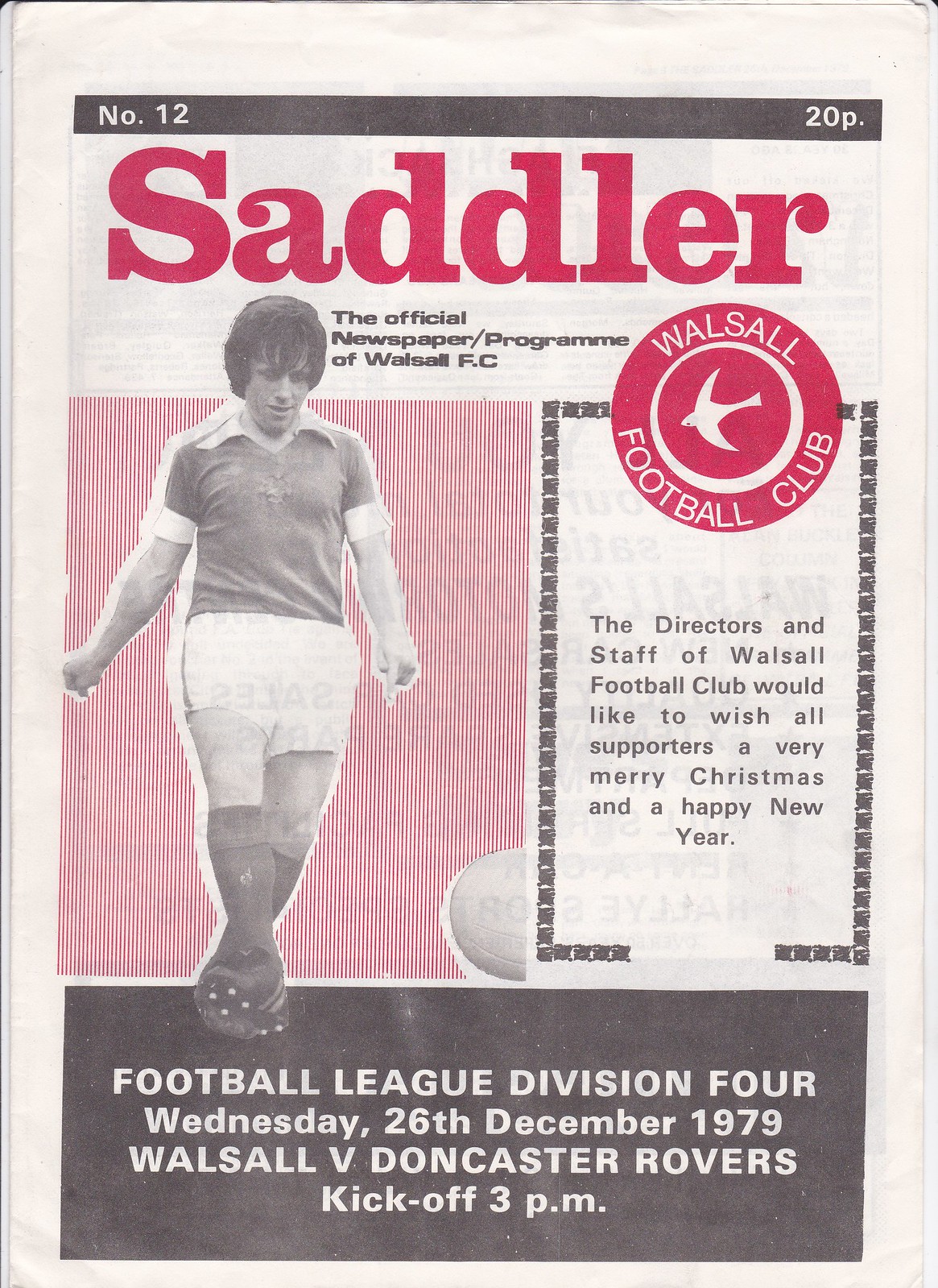This image is a faded and old soccer program pamphlet, likely from a vintage collection. The header prominently features "Number 12" indicating it's the 12th issue and the price "20 pence." Below that, in striking red letters, it says "Sadler." This signifies the official newspaper program of Walsall FC, a football club based in the United Kingdom. Additionally, there's a classic black and white photograph of a football player, who's about to kick a ball. Even though the image is monochrome, the player is depicted wearing what appears to be white shorts and a red top, enhanced by a red backdrop. Adjacent to this image is a distinct round, red logo of Walsall Football Club featuring a bird in the center. Beneath that, festive wishes from the directors and staff extend a "Merry Christmas and a Happy New Year" to all supporters. The bottom of the pamphlet, set against a gray background, details an upcoming Football League Division Four match: Walsall vs. Doncaster Rovers, scheduled for Wednesday, December 26, 1979, with a kickoff at 3 p.m.